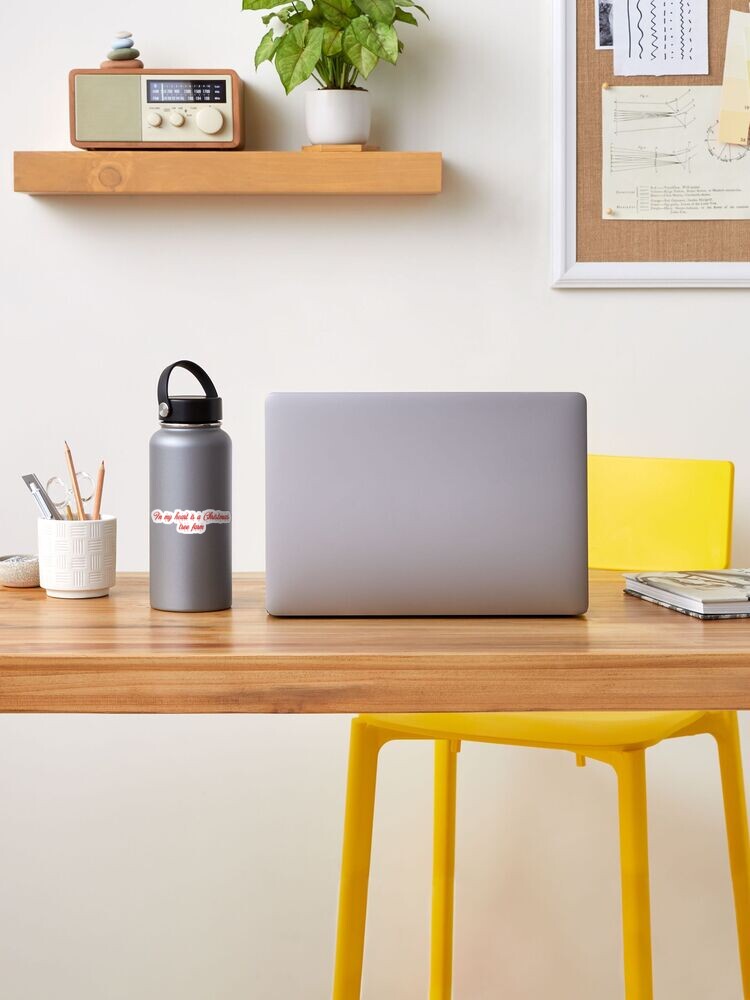The image depicts a meticulously organized, minimalist workspace set against an eggshell-colored wall. At the center of the light wooden desk sits an open silver laptop. To its left is a pink hydro flask or thermos with unidentifiable writing, and to its right, an open book or journal. A ceramic pencil holder filled with pencils, pens, scissors, and a small blade completes the desktop arrangement. The desk is paired with a yellow plastic chair, reminiscent of those found in children's classrooms, offering a simple and functional seating option.

Above the desk, a bulletin board displays various pinned notes and drawings, including graphical pieces and squiggly lines. To the left of the workspace, a wooden shelf holds an old-fashioned radio adorned with a few rocks and a green plant in a white ceramic vase, which rests on a coaster. The room is characterized by its warm tones, an absence of people or animals, and a serene, daytime ambiance that highlights the workspace's clean and organized aesthetic.